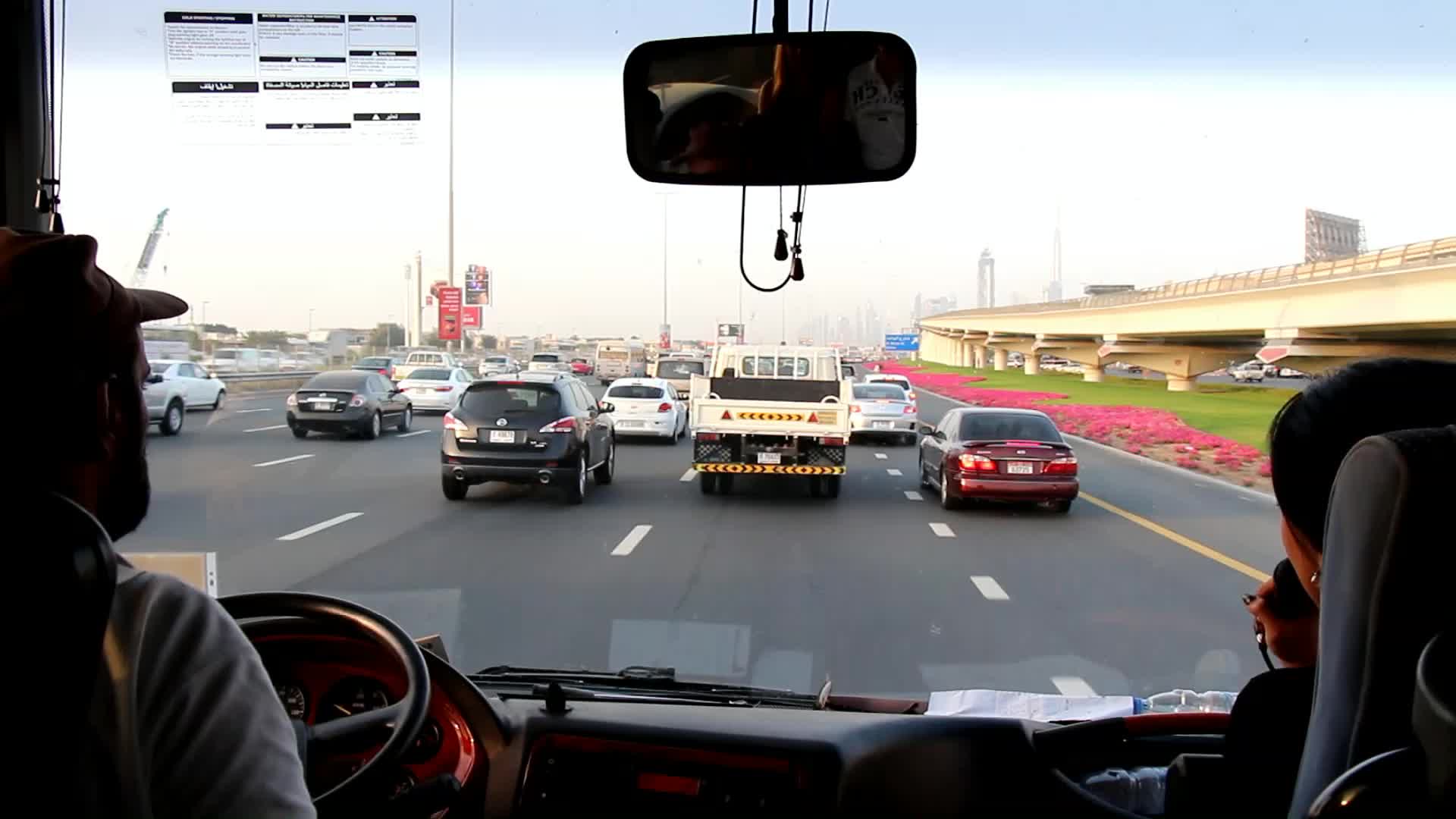This photograph captures a busy urban scene from the interior of what appears to be a large vehicle, likely a tour bus or an RV, as evidenced by the spacious windshield and overall setup. The image shows a man driving on the left side and a woman, possibly holding a microphone, seated on the right, hinting at the likelihood of a tour group. The bus is traveling on a multi-lane expressway, which has at least six lanes filled with various vehicles, including cars in black, white, silver, and red. To the right, a road bridge ramp and lush green grass adorned with pink flowers are visible, adding a touch of color to the urban landscape. The scene is set during what seems to be rush hour in a major city, as suggested by the traffic density and distant skyscrapers faintly visible on the horizon. The bus is situated in the second lane from the right, with additional road signs, light posts, and traffic moving in both directions, creating a dynamic and bustling atmosphere.